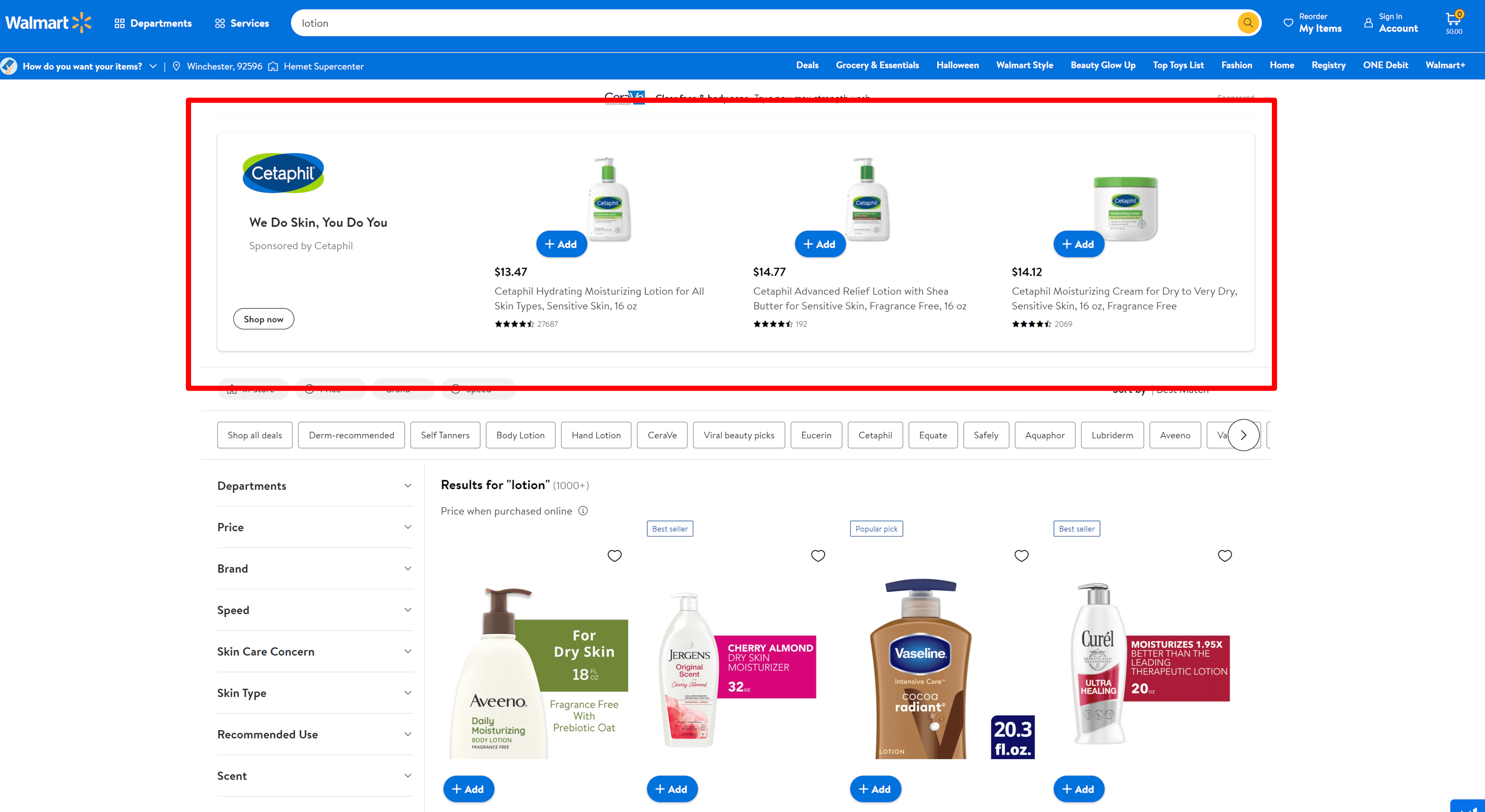Here's a detailed caption for the website screenshot of Walmart:

"The screenshot showcases the Walmart website homepage. On the left side, the distinctive Walmart logo is prominently displayed along with the word 'Walmart.' Below the logo, there are various clickable categories such as 'Departments' and 'Services.' A long search bar stretches across the top section of the page, allowing users to swiftly find products. Adjacent to the search bar, user options like 'My Likes,' 'Account,' and a shopping cart icon are visible, catering to personalized shopping and user account management.

Central to the screenshot is a red-bordered section highlighting a featured brand, Cetaphil. Within this section, the Cetaphil logo and slogan, 'We do skin, you do you,' are clearly visible, accompanied by a call-to-action button labeled 'Shop Now.' Below this, three Cetaphil products are displayed, each with a brief description, star ratings, and review counts.

On the left sidebar, various filters are listed, including 'Departments,' 'Price,' 'Brand,' 'Speed,' 'Skincare Concern,' 'Skin Type,' 'Recommend and Like,' and 'Scent.' These filters assist users in refining their product search based on specific preferences.

To the right of the Cetaphil section, additional product listings are visible. Brands such as Aveeno, Jergens, Vaseline, and Curel are displayed, with four products shown under the category 'Results for Lotion,' indicating items like moisturizing creams and lotions. The background showcases numerous greyed-out boxes with product details listed above, alongside navigation arrows for browsing through multiple listings."